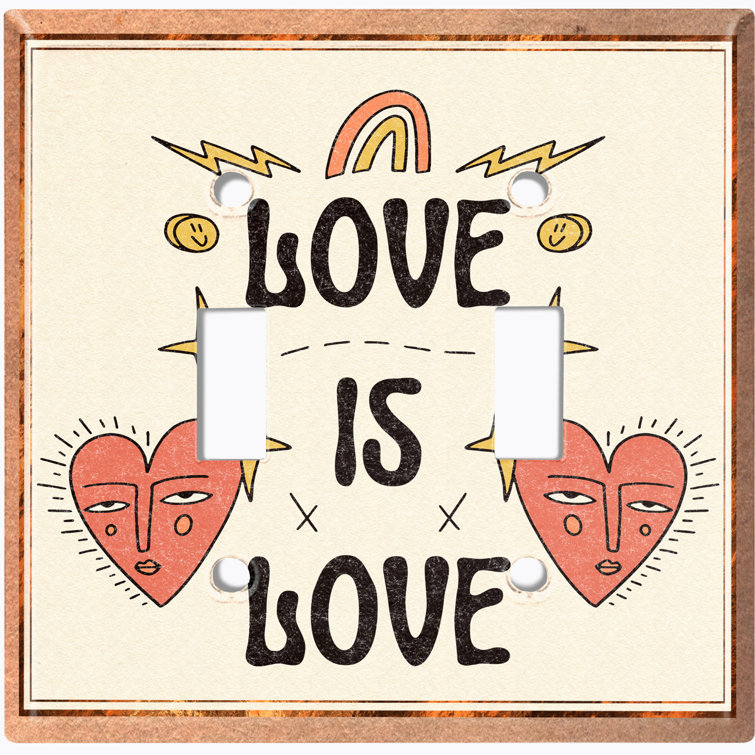This is a photograph of a framed wall hanging with a light reddish, orangish wooden border. The backdrop is very light, almost cream-colored, showcasing an animated drawing in the center. At the top of the artwork, there is a rainbow flanked by two lightning bolts—one on each side. Just beneath the rainbow, in bold black font, the words "Love is Love" are prominently displayed. Surrounding the text are two gold smiley faces on either side. Below the phrase, the poster features two red, heart-shaped characters with facial features, including eyes, a nose, and a mouth, and little black lines emanating from them. One heart on the left is shedding two tears, while the heart on the right has a yellow star sticking out from the top. Additionally, the poster includes various cutouts: two circles at the top, two circles at the bottom, and two rectangles on each side, giving the impression that it might be a decorative cover for a light switch. The entire piece exudes a whimsical and heartfelt message of love and inclusivity.